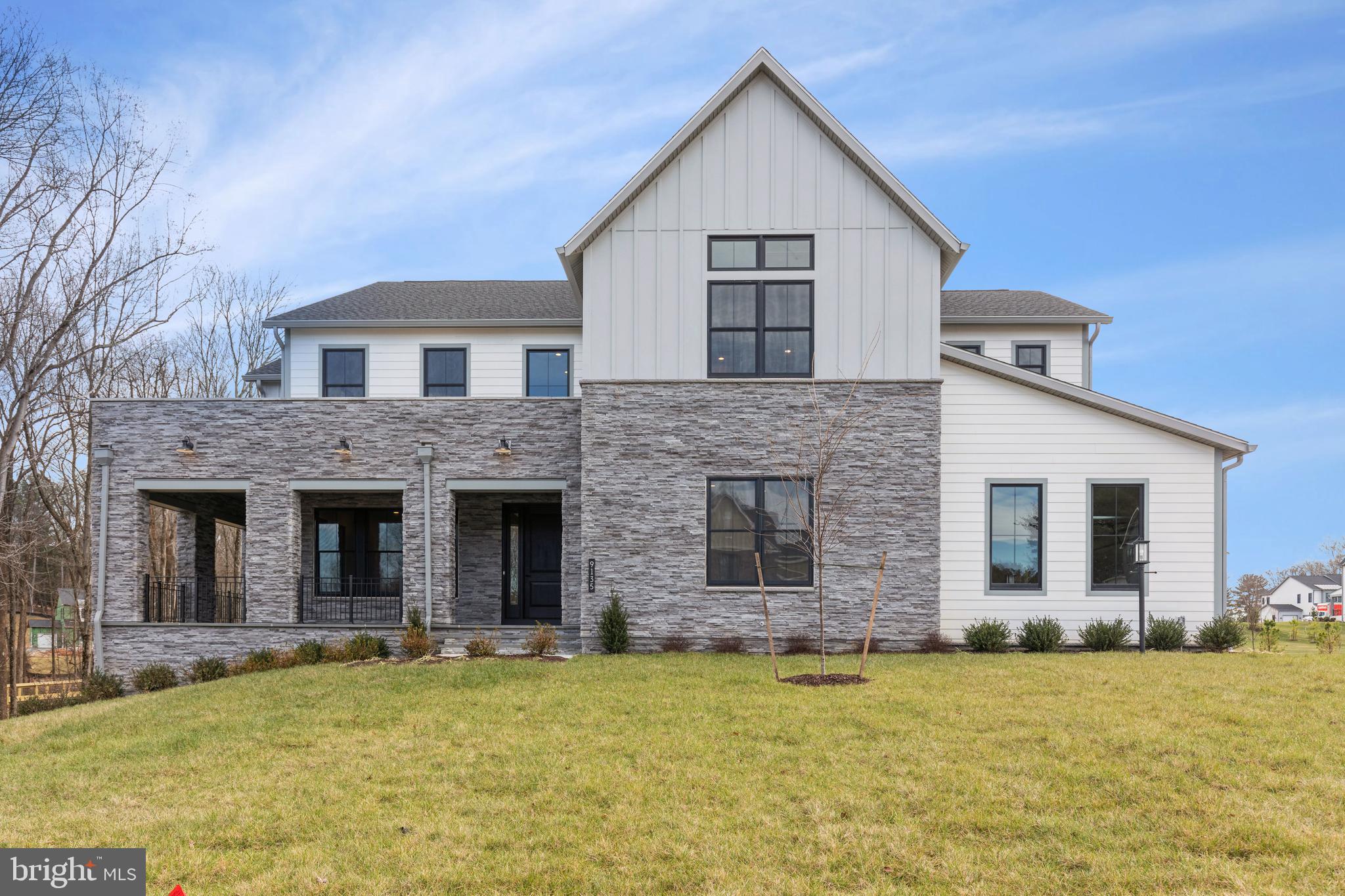This high-quality real estate listing photo showcases a large, two-story house on a slightly yellowing lawn with a recently planted, thin tree supported by two posts near the back of the lawn. The house has a distinctive two-tone exterior with a gray stone first floor that features three large openings to the left and a square window in the center. To the right side of the first floor, the house is finished in white siding with two tall rectangular windows. The second story, also finished in white paneling, has several tall rectangular windows facing the viewer. The front of the house has minimal landscaping, with a neat line of small bushes and a black fence on the deck. To the left of the image, a tree with sparse leaves can be seen, and the blue sky above features wispy white clouds. In the background, other similar type houses are faintly visible. The bottom left corner of the image displays a logo for Bright MLS.